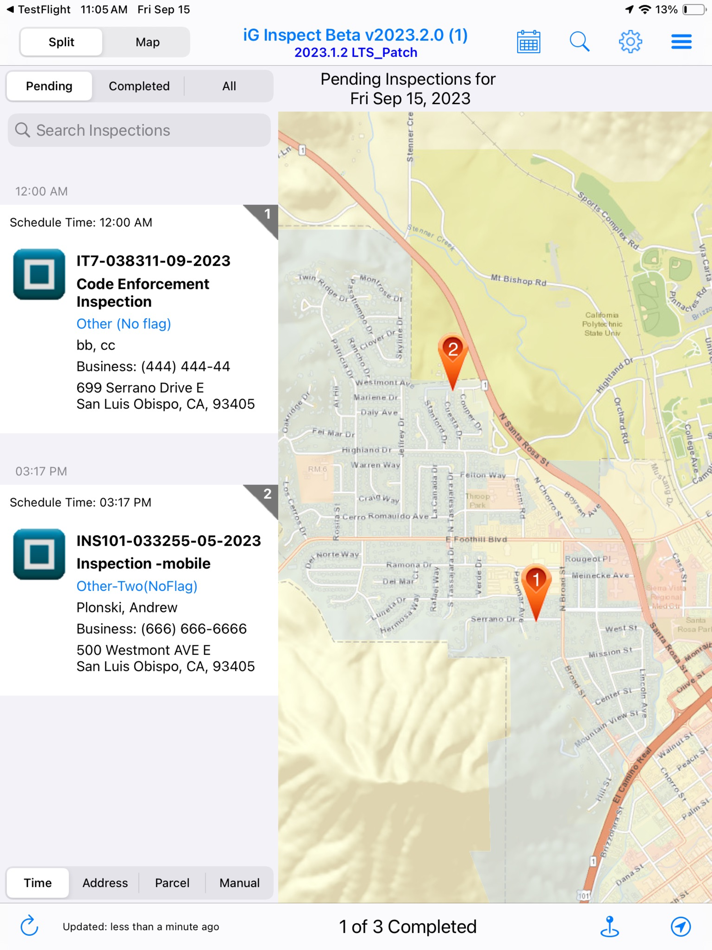A detailed screen capture from IG Inspect Beta Version 2023.2.0 displayed on a computer monitor. The interface shows a map of San Luis Obispo, California, with a focus on the area around Cal Poly and Santa Rosa Street. On the left side of the screen, there is a "Search Inspections" toolbar containing a search bar and two listed options: "Code Enforcement Inspection" and "Inspection-Mobile." These listings suggest that the software is likely used for municipal purposes, such as zoning enforcement and regulation compliance. The map view appears to be providing real-time or pre-designated inspection locations for city officials to visit or are currently inspecting.